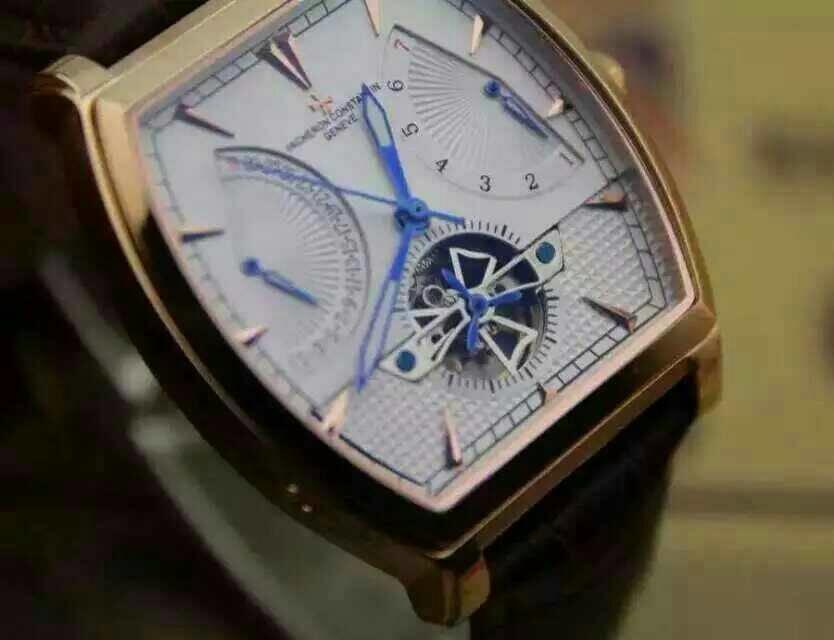This photograph showcases a close-up view of a watch face, positioned diagonally from the top left to just above the bottom right corner. The watch is encased in a slightly curved rectangular frame made of gold-colored metal. The brand of the watch is indiscernible. 

The watch face features three sub-dials. The left sub-dial, marked by a blue arrow, mirrors the right sub-dial, which also has a blue arrow and is numbered 1 through 7 in black. The central, larger hands indicate the time, with the hour hand pointing close to the 12 o'clock position, the minute hand at around 40 minutes past the hour, and the second hand near 54 seconds.

At the bottom of the watch face, there is an additional sub-dial resembling a pinwheel, adorned with a blue propeller-like design. This sub-dial displays numerous small slashes, adding to the intricate detail of the watch.